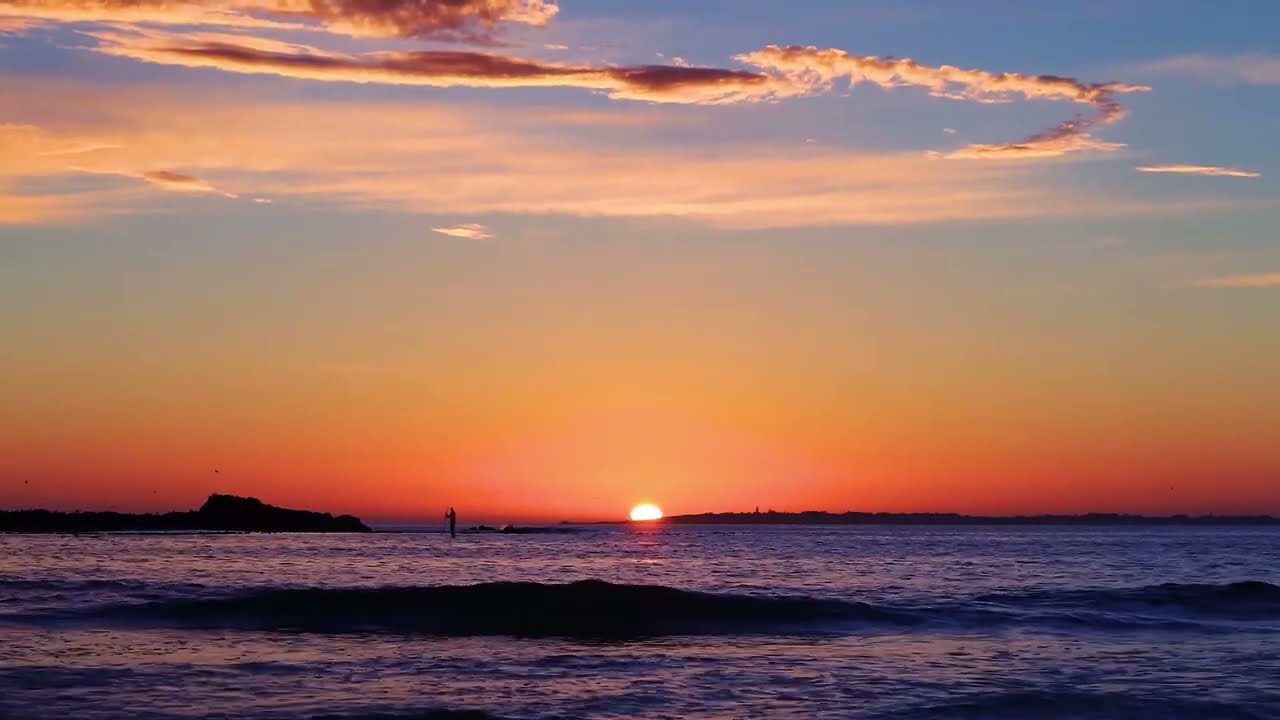The image captures a mesmerizing sunset by the ocean, with the sky painted in vibrant shades of orange, pink, and blue. At the horizon, a small, round sun is partially obscured by the calm sea, casting a warm, red hue that blends into the blue sky above. Wispy, thin clouds form rings and striations at the top of the image, adding depth to the scene. In the foreground, the water is relatively still with slight ripples, reflecting the sky's warm colors. On the left side, a low-lying landmass adds contrast to the scene. Near the center, a dark shape, possibly a rock or a wave, protrudes from the water. In the distance, slightly to the left, there's a faint silhouette of a person, possibly fishing. The overall view is serene and panoramic, capturing the majestic transition of day to night.